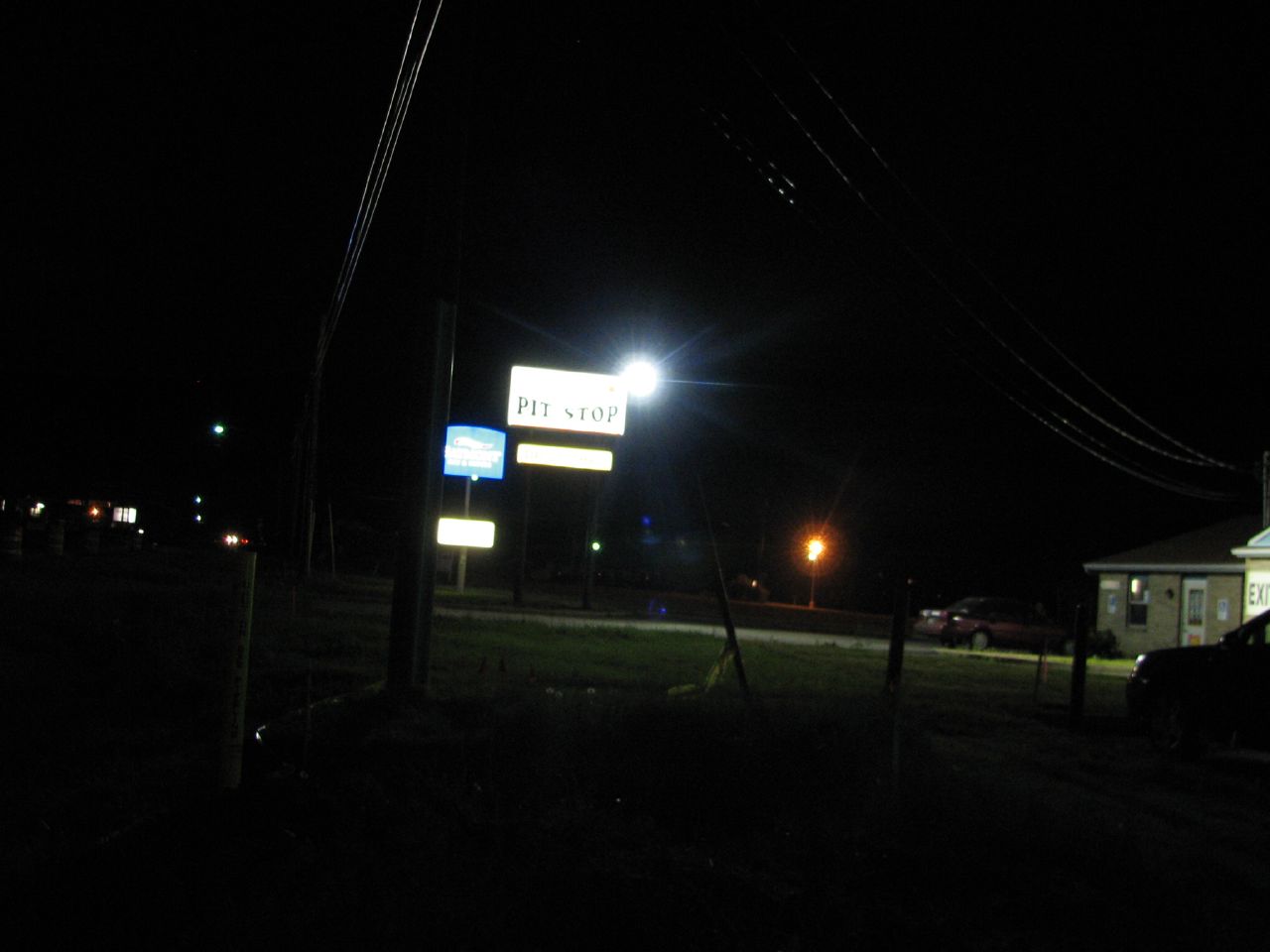This nighttime outdoor photograph captures a dimly lit scene dominated by an illuminated sign suspended on two black poles near the left of the center frame. The sign, predominantly white, features black text at the bottom that reads "Pit Stop." Below it, there is another thinner, glowing rectangular sign whose text is illegible. To the left of the main sign, a smaller blue lamp with some unreadable writing adds to the sparse illuminations. In the distance, two more illuminated signs on metal poles are faintly visible, though their details are unclear.

On the far right of the image, part of a small square brick building with a tan finish comes into view. This building includes a white door with bars across its window and an adjacent small window. A burgundy car is parked in front of this building, positioned in a three-quarter view. Additionally, the left front fender of another, all-black car is slightly visible along the right edge. Above the scene, multiple power lines crisscross diagonally from the top edge, suggesting a connection to the building.

The overall scene is enveloped in darkness, with the foreground and background almost entirely consumed by shadow. Faint distant street lights appear on the left side, providing minimal relief from the pervasive blackness.